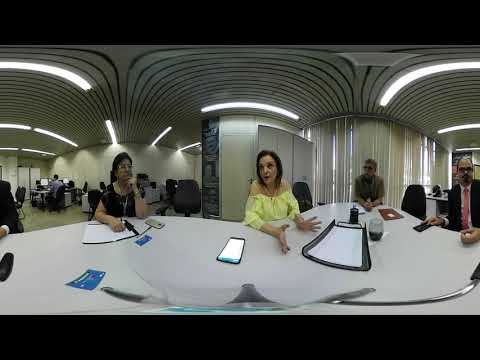In an office setting, four individuals gather around a large, irregularly-shaped white conference table. Positioned at the center is a woman in a yellow blouse, her hands open, actively speaking to the others, who are dressed in various shades of business attire. Phones, papers, and a cup are scattered across the table in front of them. Surrounding the table is a bustling office environment with people working on computers, visible through the left side of the background. To the right, a rounded window with blinds offers a view outside. The ceiling above them features three distinct geometric shapes with horizontal lines, interspersed with lights, adding a modern touch to the room. The image, taken in a 360-degree panorama, slightly distorts the scene, accentuating the dynamic atmosphere.